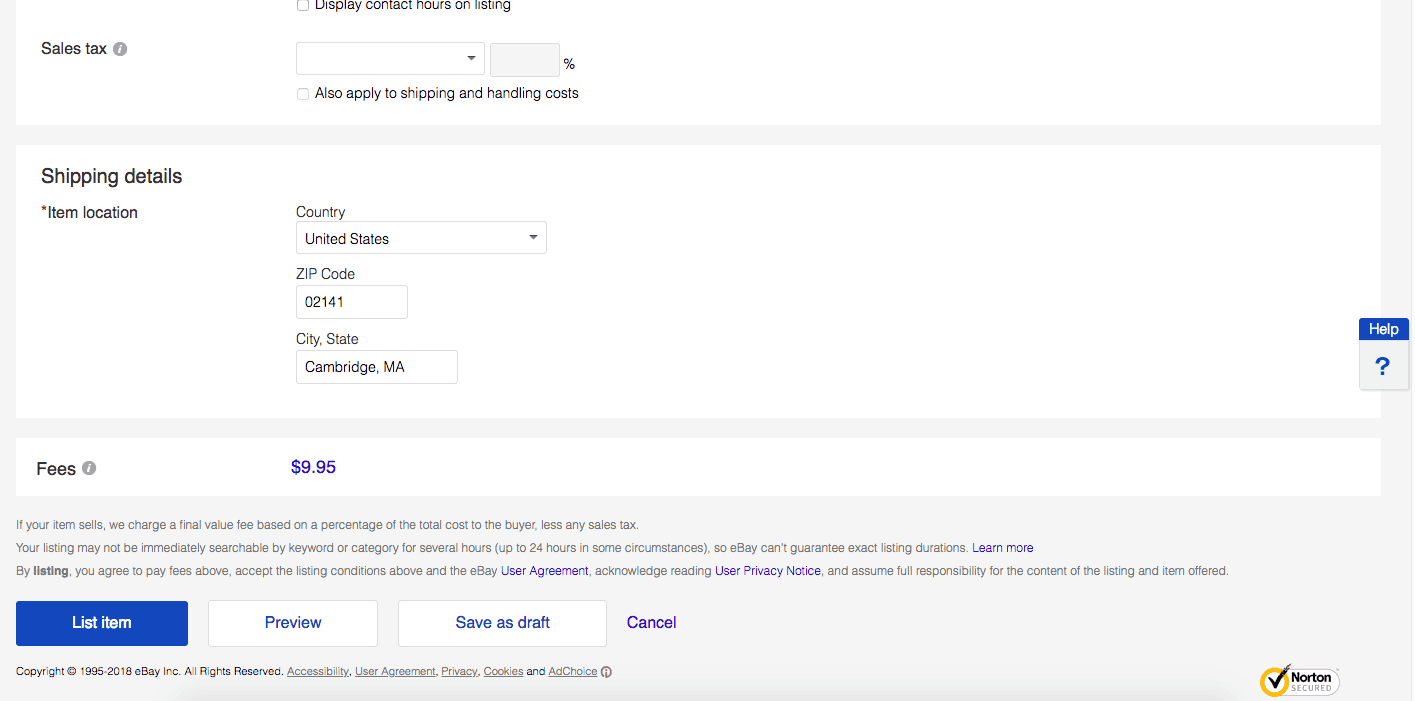The image features a user interface with a predominantly white background, partially cut off on the top part. The left side is bordered with gray, and on the right side, there is a similar gray border extending downward. The top section displays a series of black success tags with a gray circle adjacent to them, featuring a white eye icon. Below, there is a section labeled "Display Contact Arms," followed by a white rectangular box with a gray outline and a dark gray downward-pointing triangle.

Next, there is a gray rectangle displaying a black percentage value, accompanied by a checkbox. Additionally, the black text indicates involvement with shipping. A gray horizontal border separates this section from the subsequent details regarding shipping. 

Following the shipping section, there is a red "X" icon next to the text "Shipping Details," which includes fields for "Item Location," "Country" (selected as United States), "Zip Code" (entered as 02141), and "City, State" (listed as Cambridge, MA).

On the right side of the image, there is a rectangular section with a blue background at the top that contains the word "Help" in white text. Below this, the rectangle splits into a gray area with a blue question mark icon. Another gray horizontal border separates this area from the section labeled "Fees," where the fees are displayed in a bluish-purple color with a dollar sign followed by the amount "$9.95."